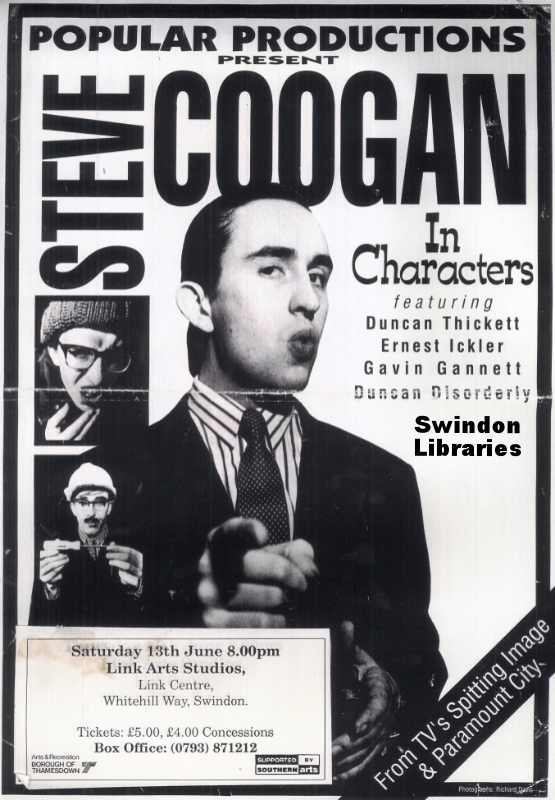This is a horizontally aligned black and white vintage advertisement, possibly from the 1970s or the 1940s. The background features a thick black border that narrows at the top, framing the image. Across the top, in bold, uppercase letters, it reads "POPULAR PRODUCTIONS" within this black border. Just below, in smaller capital letters, it states "PRESENT."

On the left side of the image, the letters of the name "STEVE" are stacked vertically in a slender font. Beside it, the name "COUGAN" appears in shorter but bolder uppercase letters. Below COUGAN, it says "IN CHARACTERS," with "IN" in uppercase and the rest in lowercase. Centered beneath this, the word "FEATURING" appears in much smaller italics, followed by the names "DUNCAN THICKET," "EARNEST ICKLER," "GAVIN GANET," and "DUNCAN DISORDERLY," each centered and in a larger font than "FEATURING."

Further down below "DUNCAN DISORDERLY," the names "SWINDON LIBRARIES" are noted in bold, centered relative to each other. 

In the bottom right corner, there is a black banner with white text that reads "FROM TV'S SPITTING IMAGE," and underneath it, "IN PARAMOUNT CITY" is centered.

The left side of the advertisement features two black and white images. The top image shows a white man in a pale or medium-colored snow cap and spectacles, leaning towards the camera with one hand on his chin, possibly holding a pacifier. The second image below depicts another white man, also in a pale snow hat with spectacles, button-up shirt, and mustache, holding his hands in front of his face with knuckles showing.

In the center left of the advertisement, a larger photo captures a man in a suit jacket with a fishnet-patterned black tie and a striped dress shirt. He has slicked-back black hair, a pale face, and is pointing directly at the viewer with pursed lips.

A white rectangular sticker with a black rectangular border is superimposed on the bottom left corner. This contains event details in a mostly bold, possibly Times New Roman, font which reads:

- "Saturday, 13th June, 8pm"
- "Link Art Studio"
- "Link Center"
- "White Hill Way, Swindon"

There’s additional information about tickets and a contact number, "Tickets £5, £4 Concessions," and "Box Office (0793) 871212," followed by an unclear block of text and a profile or italicized capital "T."

The overall setting and language suggest a British context, emphasized by the use of pounds for the ticket prices and the British spelling of "center" as "centre."